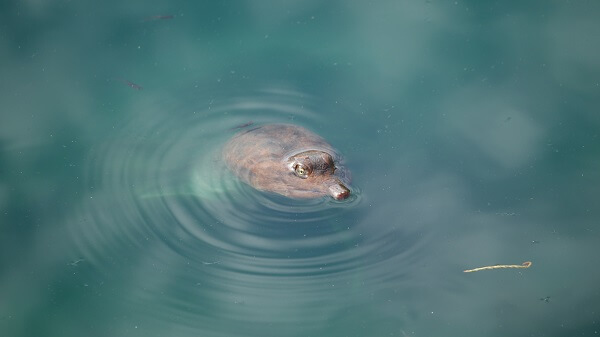This color landscape photograph captures a small brown duckling in a pond, rising up from beneath the surface. The scene is set predominantly in mottled bluish-green water, with the duckling positioned centrally and surrounded by ripples forming a circular, whirlpool-like pattern. The duckling’s head, with its rounded rectangular shape, bumpy texture, and two eyes peering up toward the viewer, barely peeks out from the water. The duckling's beak emerges partially, pointing towards the bottom right corner of the image. Additionally, a thin twig or piece of hay can be seen floating nearby. The photograph is taken from above, providing a top-down view that emphasizes the duck's mostly submerged body and the serene water texture.